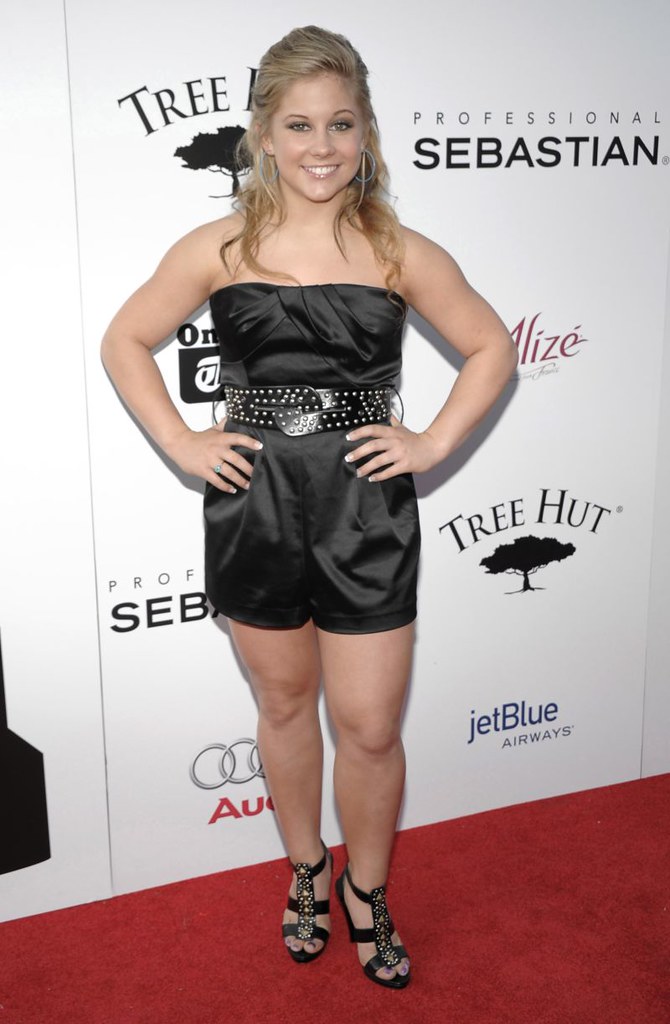In this vibrant color photograph, a young blonde woman is captured standing on a red carpet at a high-profile event. She is adorned in a stylish black ensemble, consisting of a halter top and satin shorts, accented with a clear belt featuring silver studs. Her look is elegantly completed with black strappy heels embellished with intricate detailing. With her long blonde hair pulled back, she stands confidently with her hands on her hips, smiling at the camera. The backdrop is a white wall emblazoned with various sponsor logos such as Tree Hut, Professional Sebastian, Alize, Audi, and JetBlue Airways, which enhance the celebrity glamour of the scene. The Audi logo and the red carpet add striking splashes of color to the otherwise monochrome attire. This image epitomizes the essence of a professional red carpet event, capturing both the elegance and the promotional elements seamlessly.